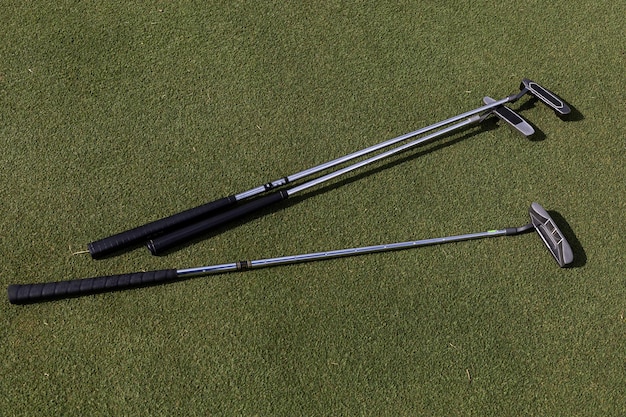The image depicts a green golf course, likely featuring astroturf due to its uniform and close-knit appearance. Three putters lie intertwined on the green grass, showcased under the bright sunlight that reflects off their stainless steel rods. The putters, each with black padded handles, exhibit silver bodies. Two of the putters are of similar length, with one shorter putter positioned underneath one of the longer ones. The long one overlaying the short one has a distinctive black head, while the shorter one features a silver head. Off to the bottom of the image, another putter with a textured silver head is positioned almost horizontally, its right side slightly elevated, and together, the arrangement of the putters forms a narrow V shape.